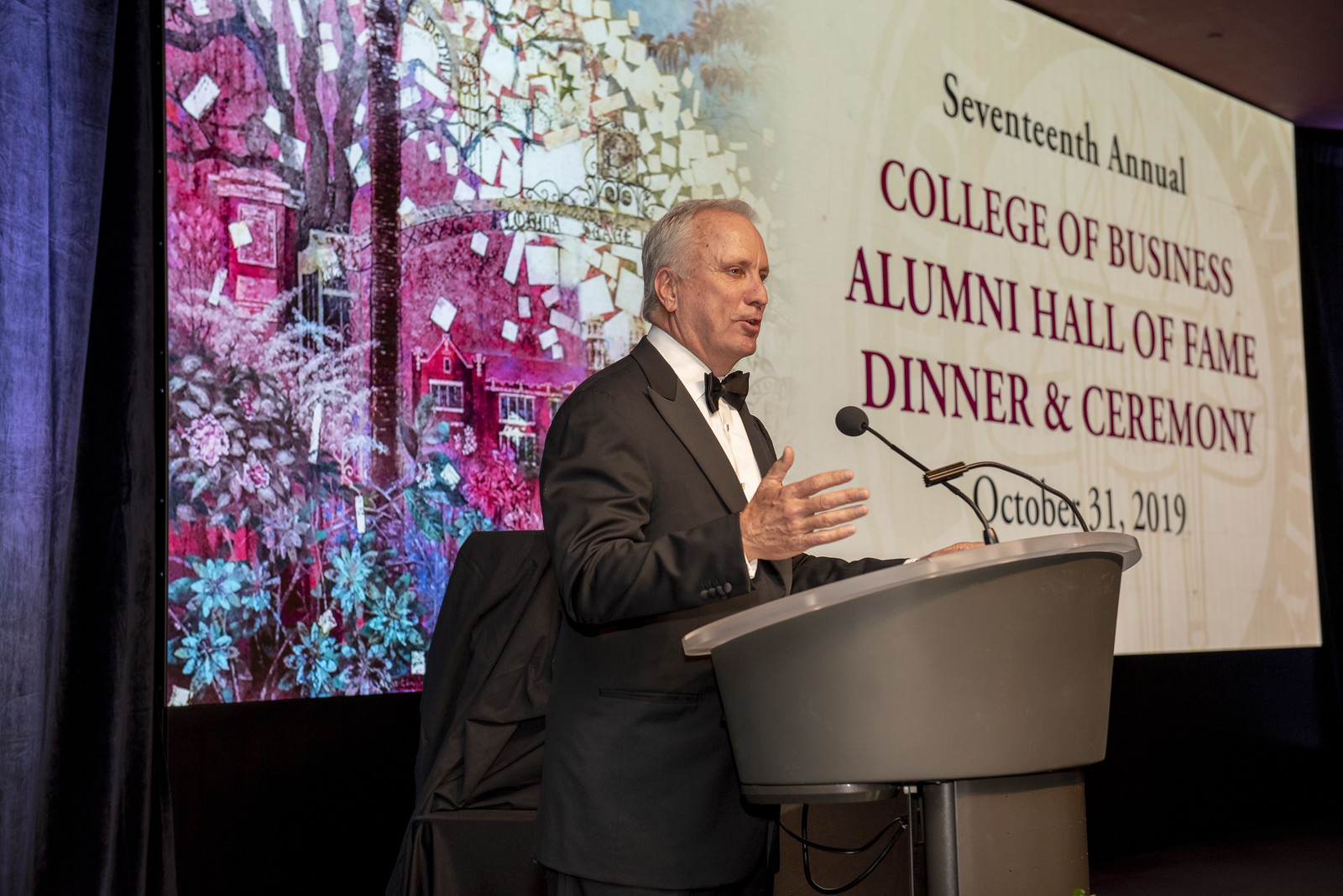In the center of the image, an older white man, likely in his late 50s to early 60s, is standing at a podium with a silver slanted top and two microphones. Dressed in a tuxedo with a bow tie, he is actively addressing a crowd with his right hand raised, thumb up and fingers pointing towards the audience, a typical gesture for emphasizing points during a speech. The backdrop features a projected artistic banner that reads "17th Annual College of Business Alumni Hall of Fame Dinner and Ceremony, October 31, 2019," against a backdrop reminiscent of watercolor-painted buildings in reddish-pink hues with blue, pink, and purple flowers, and papers seemingly flying from rooftops. The setting is indoors with surrounding colors of purple, pink, gray, light blue, tan, maroon, black, and brown, adding to the formal and ceremonial atmosphere of the event.